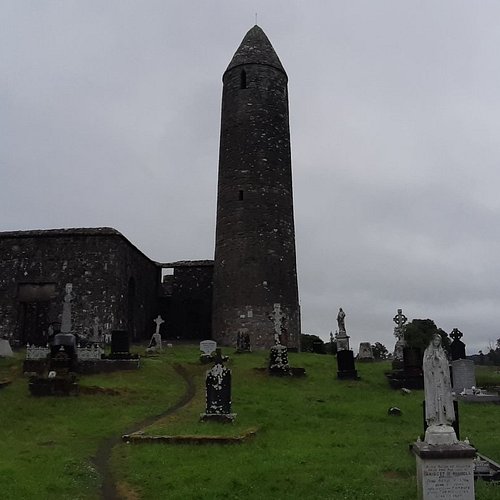The image captures an outdoor scene on a hill with a historic, eerie ambiance. The overcast sky is dominated by grey clouds with a hint of blue peeking through, casting a somber light over the landscape. In the background, a dark grey stone tower resembling a silo or a weathered castle turret rises into the sky, topped with a weather vane and transitioning to a lighter grey at its base. Adjacent to this tower is a connected flat, box-like structure made of similarly aged grey stones. The foreground features a grassy hill dotted with an array of gravestones, some adorned with crosses and figurines, including a notable white stone statue of the Virgin Mary. The markers range from grey to black, with some displaying patches of light blue mold. A narrow dirt trail meanders up the hill towards the historic buildings, encapsulating the scene in an almost spooky atmosphere of antiquity and reverence.